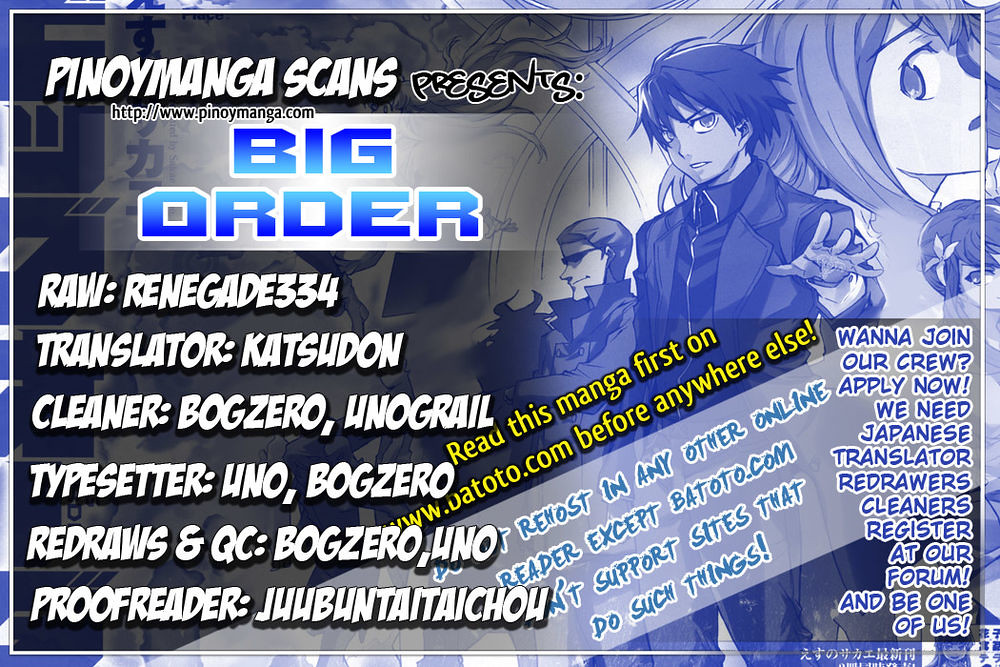The digital advertisement showcases a vibrant, multi-colored banner from Pinoy Manga Scans for their manga project titled "Big Order." The primary colors are blue and white with some shades of gray, surrounded by a blue border. The background features three artistically drawn anime characters: a person on the left wearing sunglasses, a middle figure with his body slightly turned and head facing the viewer, and the head of a young girl positioned in the upper right corner. The textual part of the advertisement lists credits for the contributors: RAW by Renegade334, translation by Katsudon, cleaning by BogZero and UnoGrail, typesetting by Uno and BogZero, redraws and quality control (QC) by BogZero and Uno, and proofreading by Jubun Taintei Chao. On the right side, it prompts readers to join their crew by applying for positions like Japanese translators, redrawers, and cleaners, directing them to register at their forum. Additionally, the ad emphasizes that the manga will be available first on Batoto.com and warns that using other sites undermines their distribution goals. The overall design and characters strengthen the appeal of this project, making it an engaging call for participation and readership.